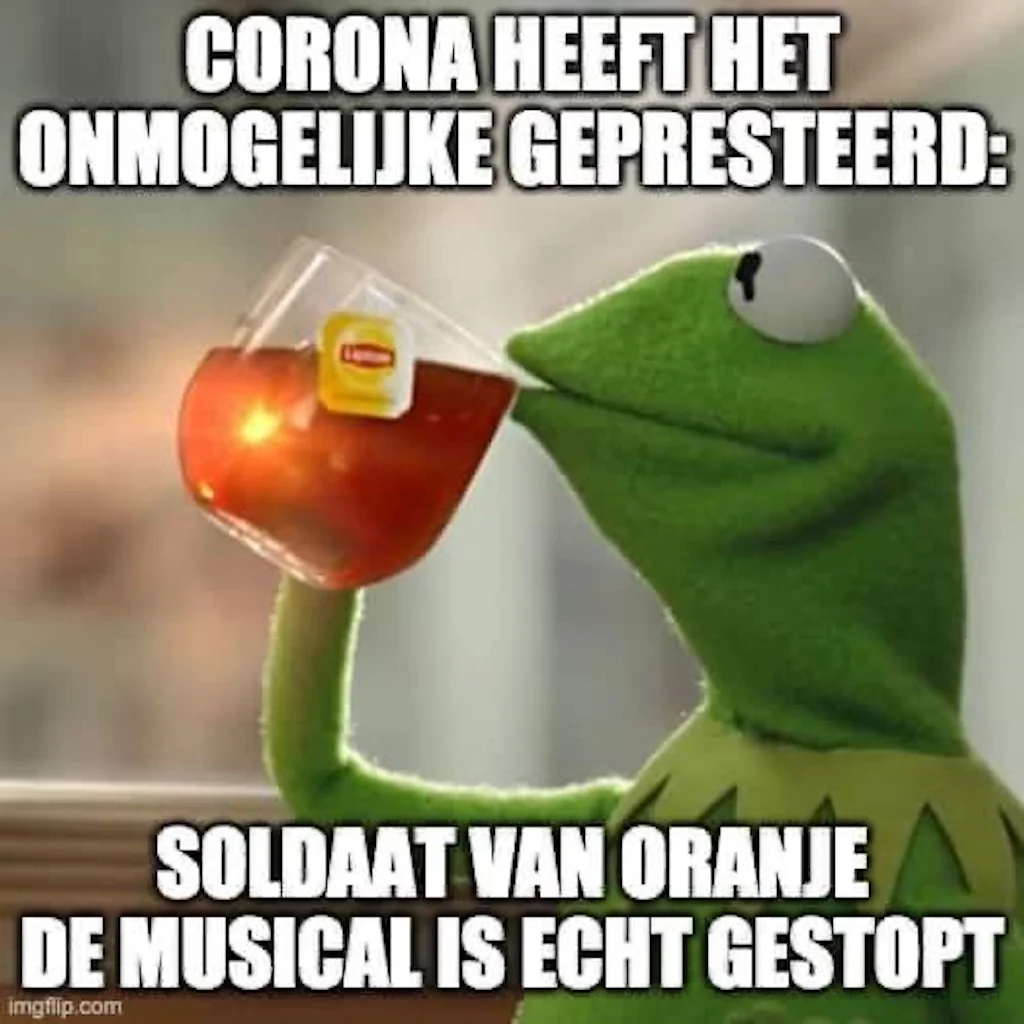The image is a meme featuring Kermit the Frog, the iconic green character from the Muppets, holding a clear glass cup with Lipton tea. Kermit, with his distinct white eyes featuring little black pupils, is sitting on what appears to be a wooden bench with one arm resting on the back. He is facing to the left. The image has white, bold text at the top that says "Corona," while additional text in an unknown language appears below, all in typical meme style. In the bottom left corner, the meme is credited to ImageFlip.com. The background behind Kermit is significantly blurred, making it indistinguishable. The Lipton tea tag is visible but blurred enough that the red and yellow label isn't fully legible.